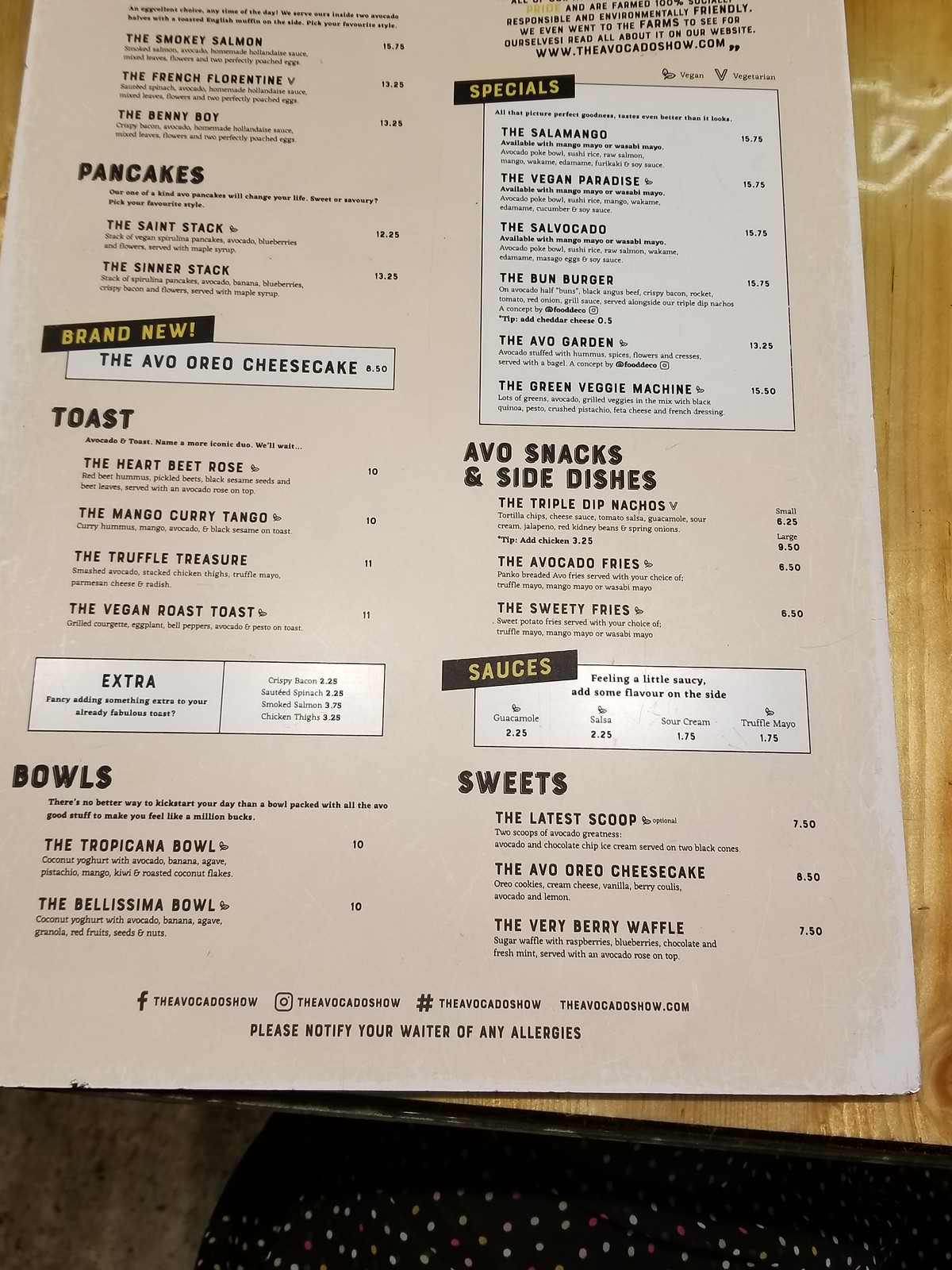This photograph captures an ivory-colored menu, meticulously organized with categories such as pancakes, toast, bowls, sweets, apple snacks, and side dishes. The menu features several white boxes outlined in black that highlight the specials and new items. Among the specials is the intriguing avocado Oreo cheesecake, while the sweets section boasts the latest scoop. The bowls include options like the Bellissima bowl and the Tropicana bowl. Other tempting menu items listed are avocado fries, mango curry, mango curry toast, the center stack of pancakes, and the saint's stack of pancakes, along with a selection of sandwiches. The clean layout and contrasting colors make the menu easy to read and visually appealing.